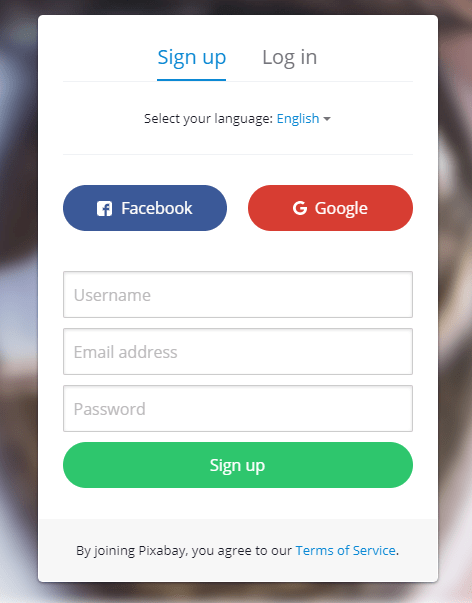This detailed caption clarifies and organizes the information for better readability:

"A screenshot depicts a sign-up and log-in window with a clean, white background. At the very top, in bold blue text, it says 'Sign Up,' accompanied by a blue underline. To the right, the 'Log In' option is displayed. Beneath these options, there's a section labeled 'Select your language,' showing 'English' in blue text with a downward-facing arrow beside it for language selection.

Below the language selection, there are two prominent buttons: the first is a Facebook sign-up button with a navy blue background, and the second is a red button labeled 'Google.' Following these buttons are three input fields for 'Username,' 'Email Address,' and 'Password.'

Underneath the password field, a green 'Sign Up' button invites users to complete their registration. At the footer of the pop-up window, there is a section with a light gray background. In this section, black text indicates, 'By joining Pixabay, you agree to our Terms of Service,' where 'Terms of Service' is a clickable hyperlink."